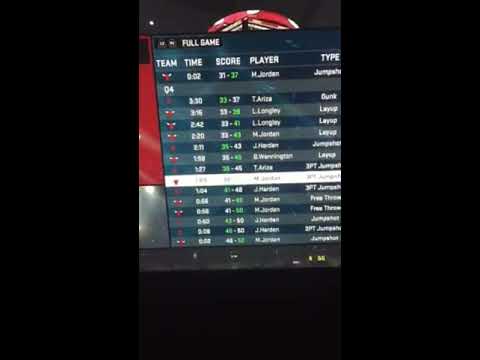The photograph captures a digital display screen, possibly from a TV or a computer, featuring a scoreboard with predominantly black, blue, and gray hues. The scoreboard, titled "Full Game" at the top left, lists columns labeled "Team", "Time", "Score", "Player", and "Type" in white text. The rows on the scoreboard are color-coded with alternating blue and gray backgrounds, and the text across these rows is mostly in white with some numbers highlighted in green. One specific row stands out with a white highlight on the left side. In the background, the display has a black surface with two prominent vertical black strips flanking either side of the screen. The image appears slightly angled, and it remains unclear whether it was taken indoors or outdoors or if it’s a real photo or digitally created. Despite some blur, the red and white objects on the screen are visible, contributing to the overall color scheme.